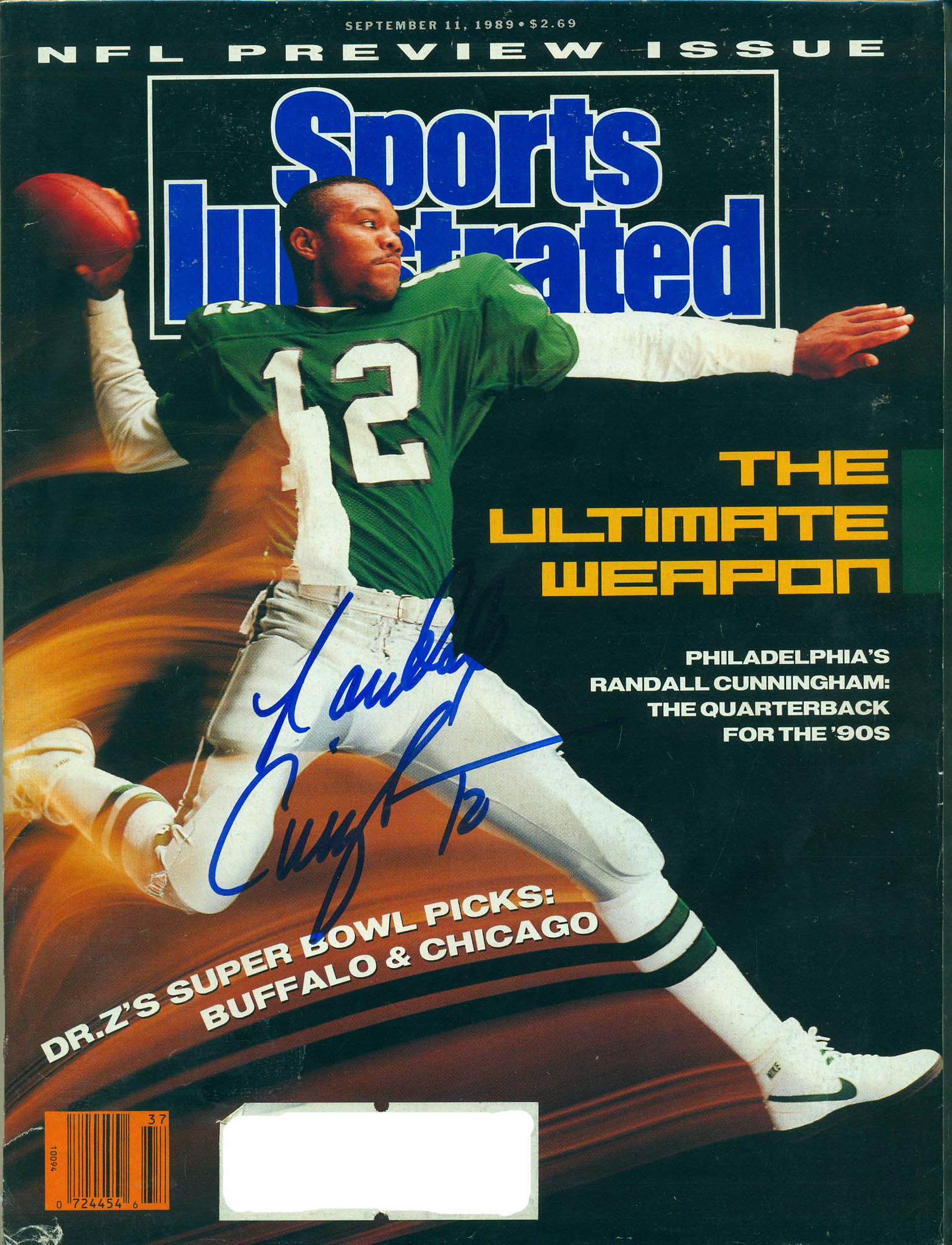This is the cover of the September 11, 1989 issue of Sports Illustrated, priced at $2.69. The white font at the very top reads: "September 11, 1989," flanked by "Sports Illustrated" in a thin white-bordered box with blue lettering. Below, in spaced letters across the page, is the headline "NFL Preview Issue." Centered on the cover is a dynamic image of Randall Cunningham, the Philadelphia Eagles' quarterback, mid-air in a classic Heisman pose. Wearing a green jersey with the number 12 and black-outlined white numbers, Cunningham clutches a football in his bent right arm, with his left arm extended straight out. He pairs his jersey with white long sleeves underneath, white pants, and white knee-high socks that have two black stripes near the top. His white Nike shoes feature a black swoosh and rubber soles. A white towel tucked into his belt flutters behind him as he moves, creating a sense of motion. 

In a yellow, computerized font to Cunningham's right are the words, "The Ultimate Weapon." Below this, in white block lettering, it reads, "Philadelphia's Randall Cunningham: The Quarterback for the '90s." An orange motion blur trail highlights the player's dynamic movement, with white lettering inside that reads, "Dr. Z's Super Bowl Picks: Buffalo and Chicago." The cover's hunter green background complements Cunningham's jersey, and a black-barred barcode and a white mailing address box are located at the bottom. An autograph in blue sharpie adorns the cover, contributing to its collectible appeal.